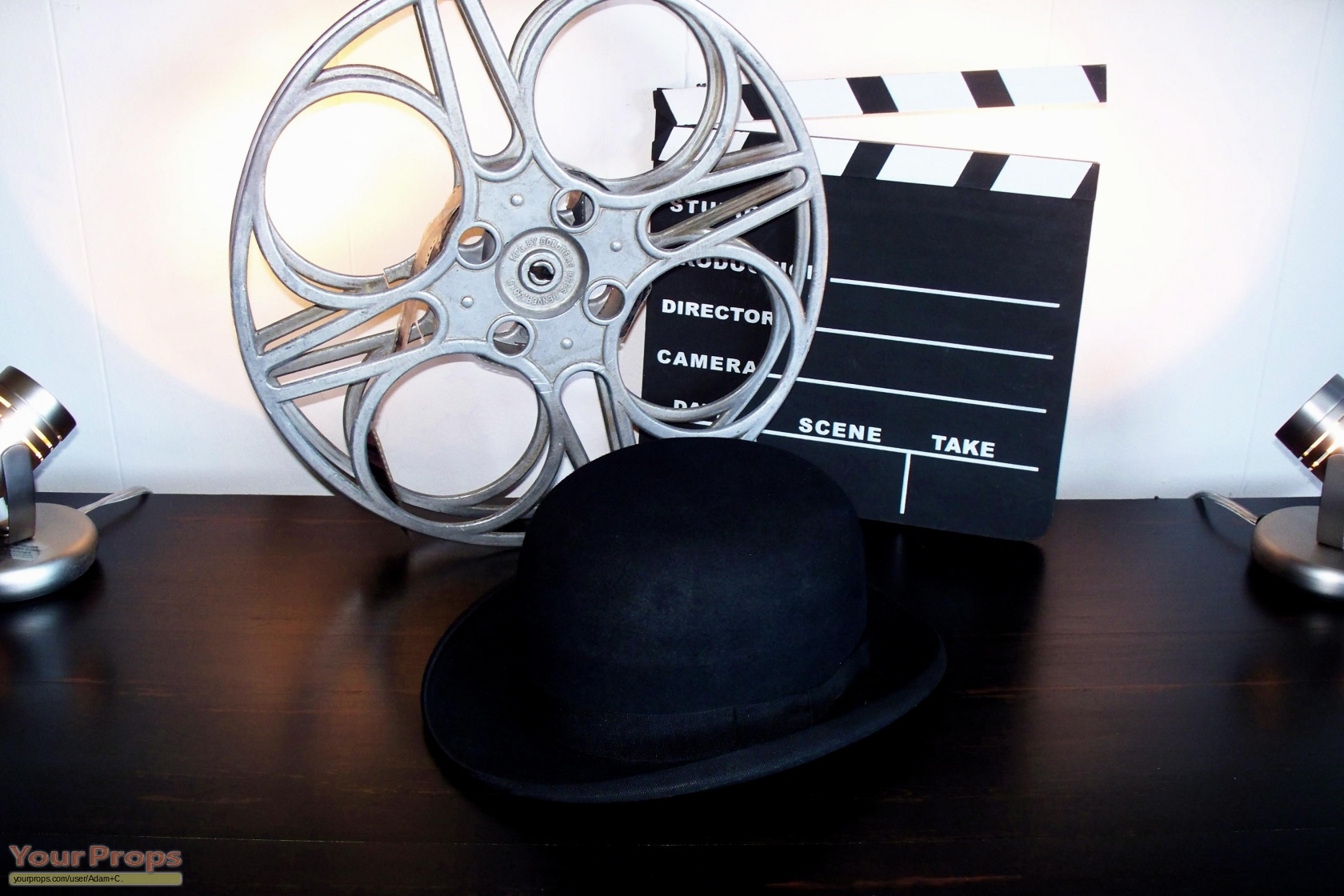This indoor photograph showcases a staged scene with a white wall background. Central to the composition is a dark brown wooden table adorned with several vintage movie props. Dominating the table is an empty silver movie reel, positioned next to a classic black bowler hat. To the right of these, there is a traditional black and white director's clapboard, complete with fields for scene, take, camera, and director, but left blank for manual entry. Flanking the setup on both the left and right sides are two silver spotlight lamps, casting a bright white light towards the center of the display. In the bottom-left corner of the image, an orangish watermark reading "yourprops" can be seen, accompanied by a small, hardly legible yellow box with additional text, identifying the website yourprops.com/user/Adam+C. This meticulously arranged photograph effectively highlights iconic filmmaking props, evoking a sense of classic movie production.